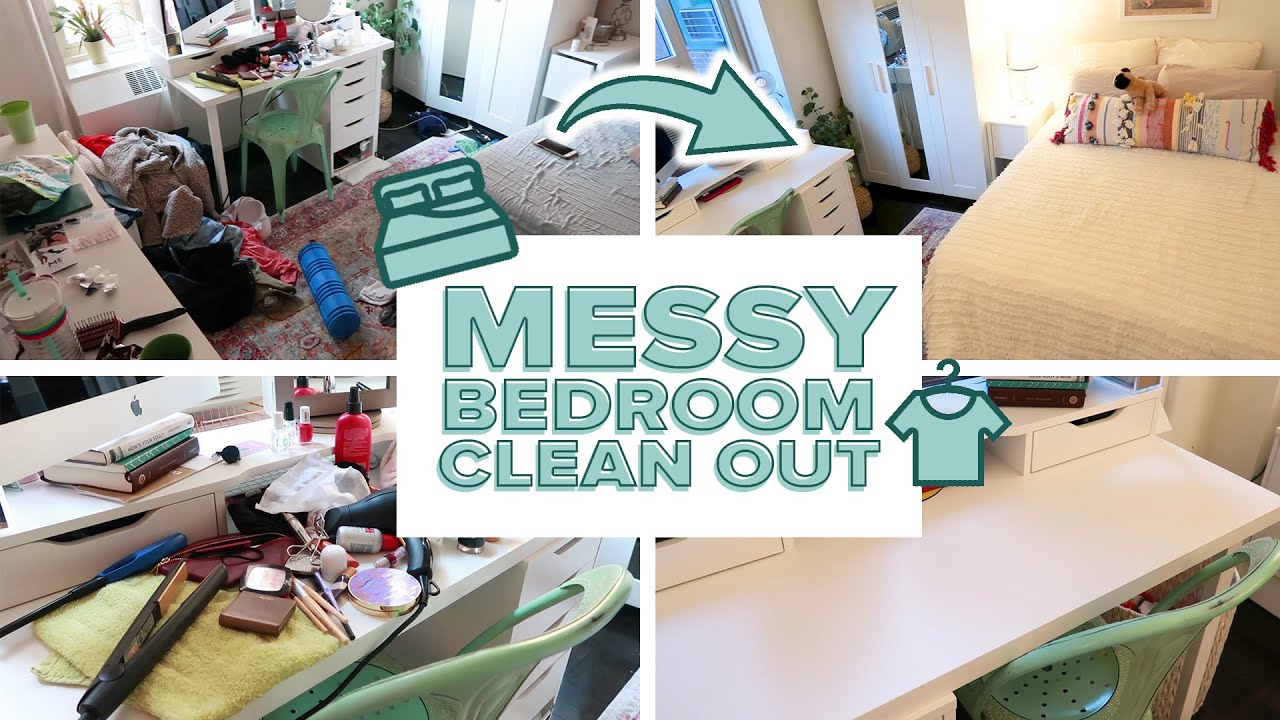The image serves as an advertisement or guide for cleaning a messy bedroom, showcasing a transformation through detailed before-and-after photographs. The center of the image features a white text block with mint green letters that say "Messy Bedroom Cleanout," accompanied by a cartoon bed at the top and a cartoon shirt on a hanger to the right. An arrow above this text block directs attention from left to right, indicating the transition from mess to cleanliness.

The main image is divided into four quadrants with white space between them. The upper left quadrant displays a cluttered bedroom featuring a dresser and a vanity mirror, with items scattered everywhere including makeup, exercise equipment like a foam roller or yoga mat, clothing, and hairbrushes. The lower left quadrant provides a close-up of the messy vanity, showing an assortment of items such as a flat iron, an Apple monitor, books, makeup, and toiletries.

On the right side, the upper right quadrant reveals the transformed bedroom, with a neatly made bed adorned with colorful throw pillows and a tidy space. The lower right quadrant focuses on the now-clean desk, presenting a serene, white, and organized workspace.

Overall, the image highlights the significant improvement achieved through cleaning and organizing, moving from chaotic disarray to neat order.